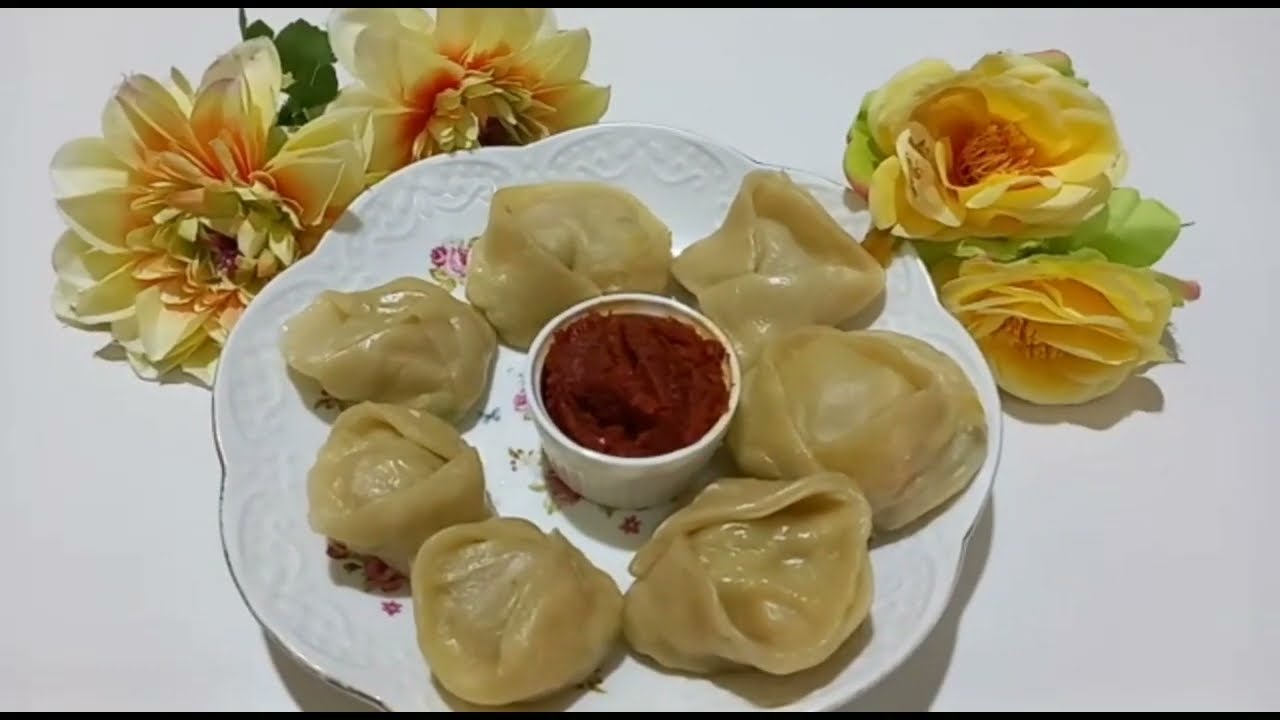The horizontal rectangular image, bordered by thin black lines at the top and bottom, features a white plate with an intricately carved floral design on the edges. The plate is garnished with vibrant decorations and holds seven dumpling-like or pierogi-like items arranged around a small, round white container filled with red sauce, possibly marinara. Beneath the dumplings, partially visible are purple and pink flowers adding bursts of color to the plate. Outside the plate, on the white table surface, there are four yellowish flowers with sprinklings of orange on their insides; two positioned on the upper left and the other two on the upper right, each accompanied by deep green and lighter green leaves. The overall presentation is elegant and carefully composed, highlighting vibrant colors and a well-structured arrangement.